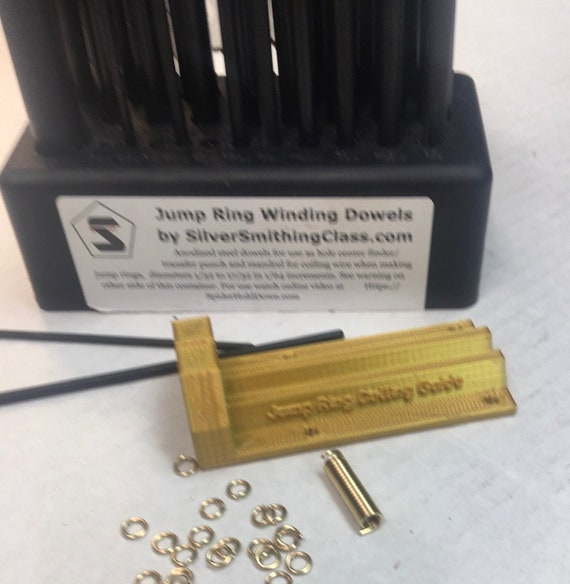The image showcases a piece of silversmithing equipment with a label that reads "Jump Ring Winding Dowels by Silversmithingclass.com." The device, primarily black, features numerous black poles extending upward from a rectangular base. In front of the base is a golden tool, labeled "Jump Ring Cutting Guide," with two rails extending to the right and a block on the left-hand side. Scattered around the guide are numerous small golden rings, both individually and coiled together. Additionally, two thin black rods are positioned on the same surface as the rest of the equipment. The label on the equipment includes a black S logo inside a pentagon and several lines of text below, though they are illegible due to the image's blur.